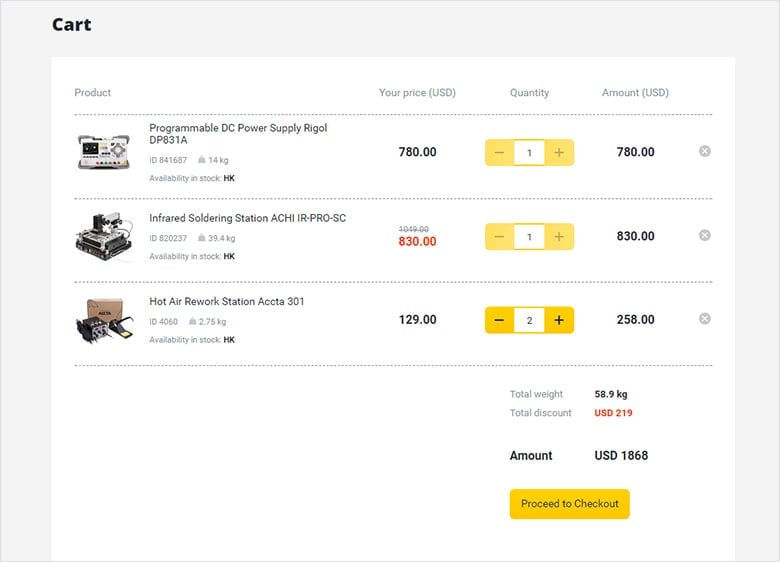**Detailed Screenshot Description:**

The image is a landscape screenshot, likely taken from a laptop screen. It showcases a shopping cart interface with a predominantly dark gray background enveloping the screen from the upper left and top left to the lower left and right corners. The central portion of the interface features a distinct white section.

In the upper left-hand corner, there is text that reads "Cart."

Within the white section, there are four rows, organized into multiple columns. The first column header, in a very light gray font that is hard to read, is labeled "Product." Below this header, each row contains an image of the respective product accompanied by its title:

1. **First Row:** Displays the image and title "Programmable DC Power Supply, RIGOL."
2. **Second Row:** Shows the image and title "Infrared Soldering Station, ATHI."
3. **Third Row:** Presents the image and title "Hot Air Rework Station, ACCTA."

The next column is labeled "Your Price in US Dollars" and lists the price for each item:
- For the "Programmable DC Power Supply, RIGOL," the price is $780.
- For the "Infrared Soldering Station, ATHI," the price is $830, marked in red indicating a sale price reduced from $1049.
- For the "Hot Air Rework Station, ACCTA," the price is $129.

The subsequent column allows for the addition of product quantities:
- Quantity 1 for the "Programmable DC Power Supply, RIGOL."
- Quantity 1 for the "Infrared Soldering Station, ATHI."
- Quantity 2 for the "Hot Air Rework Station, ACCTA."

The final column shows the total price for the selected quantities of each product:
- $780 for one "Programmable DC Power Supply, RIGOL."
- $830 for one "Infrared Soldering Station, ATHI."
- $258 for two "Hot Air Rework Station, ACCTA."

At the bottom right-hand corner, there's a summary indicating the total weight of the products as 58.9 kilograms. The total discount applied is $219, resulting in a final amount of $1868 in US dollars. Below this information, a yellow button labeled "Proceed to Checkout" is prominently displayed.